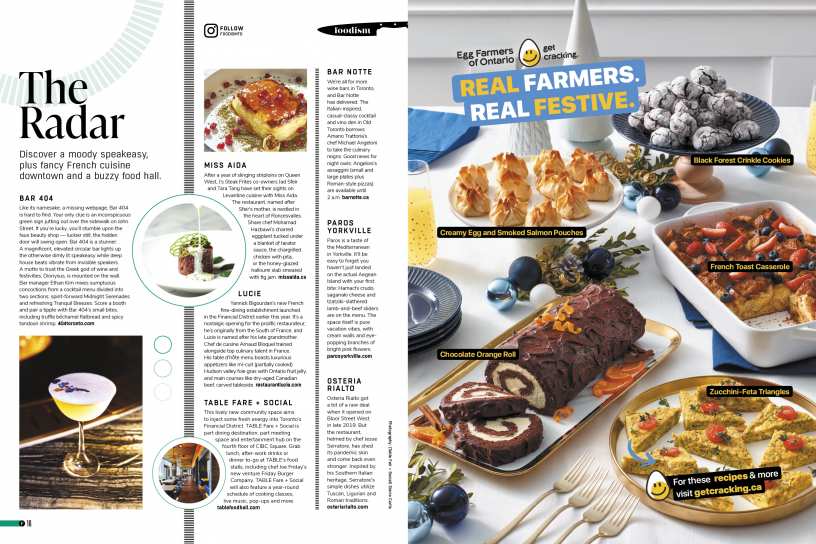In the image, a moody speakeasy ambiance is juxtaposed with fancy French cuisine in an urbane downtown setting, complemented by the buzz of a trendy food hall named R404. An article highlights these sophisticated culinary offerings with visuals, including one featuring a cocktail served in a champagne glass, and the name “Miss AIDA.”

Besides, there is mention of venues like “Lucy” and “Lucie Table Fare Social Bar,” and notable tags like “Notte Pards” in the Yorkville area, as well as “Rialto.” To the right, a photograph captures an abundant spread on a white tablecloth. The arrangement promotes the “Real Farmers, Real Festive” campaign by the Egg Farmers of Ontario, encapsulated in a blue, red, yellow, and white font theme. 

The dishes showcased include "Creamy Eggs and Smoked Salmon Pouches," "Black Forest Crinkle Cookies," "French Toast Casserole," and "Zucchini Feta Triangles." Each delicacy is tagged with black rectangles featuring text in yellow font. The text at the bottom of the image directs viewers to “GetCracking.ca” for these festive recipes and more culinary inspiration.